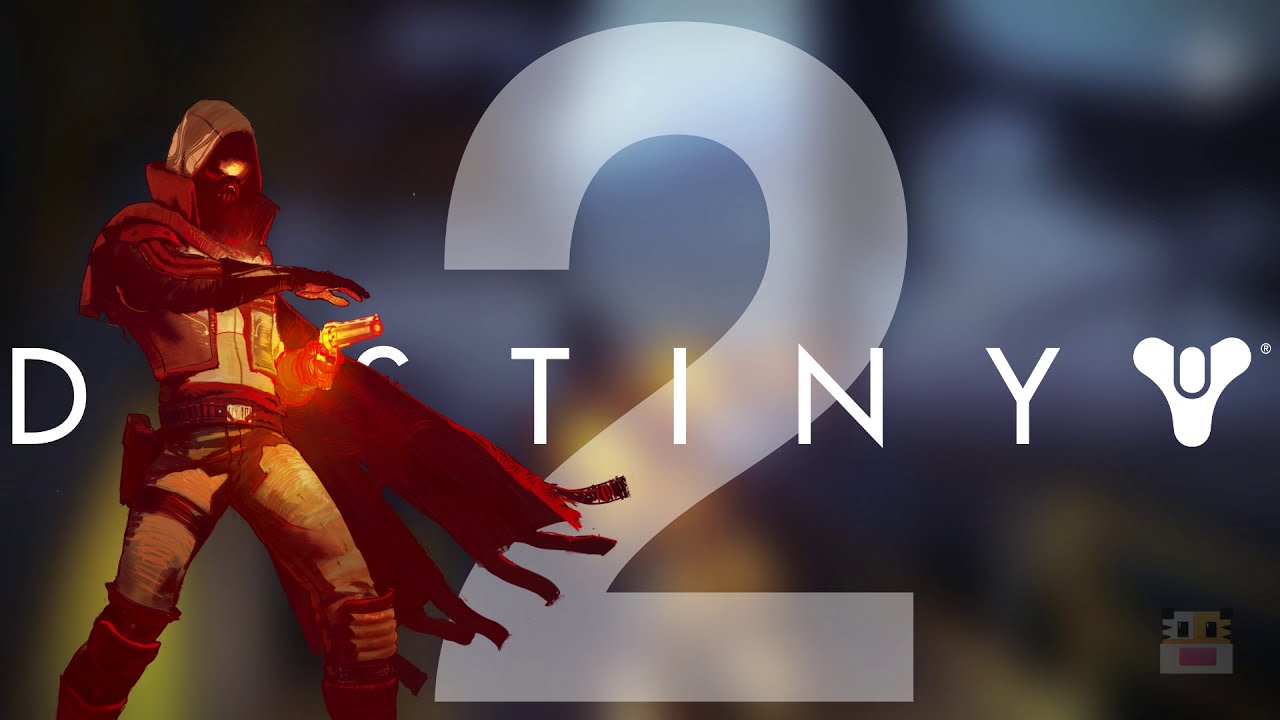The image appears to be a detailed screenshot from the video game "Destiny 2." Dominating the center is a large, washed-out whitish-gray number "2," which fills most of the background. The background itself transitions from a dark, blurry grayish-blue color in the top two-thirds to a yellowish glow in the bottom third.

On the left side of the image, a male character is positioned from the shins up. He is adorned in a red-toned, high-collared vest over a jacket with a hood. His face is partially obscured by a mask, except for a gold-lit nose, sharp teeth, and a single orange beam between the eyes, suggesting illuminated facial features. The character's right arm is extended forward, bent at the elbow, while his left arm, tucked closer to his side, wields a glowing, light-emitting yellow revolver aimed cowboy style, ready to fire. His attire includes gray pants with items strapped around his waist and leather gloves. Additionally, he has a cape flowing towards the right side of the screen.

Mid-image, the word "DESTINY" extends horizontally across the scene, partly obscured by the character. The "D" starts on the left, visible to the left of the character, while the letters "E" and "S" are obscured, continuing with "TINY" spread towards the right. To the right of the text is a distinctive Y-shaped symbol with circular tips and a round-edged vertical rectangular cutout. In the lower right corner, a logo resembling a tiger face within a square punctuates the composition.